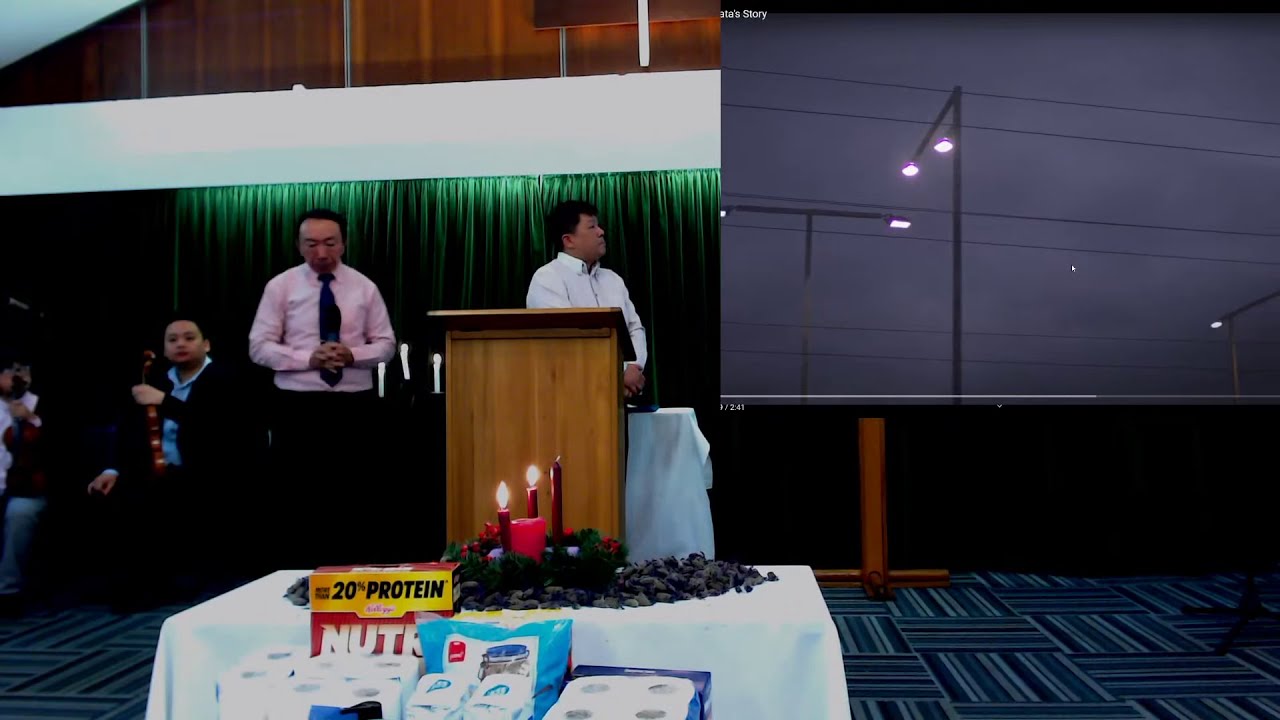The image captures a solemn indoor gathering set in an elegant community space, possibly a church or a venue for a significant event. The setting features a sloped wooden ceiling, above which hangs a backlit panel of green curtains. At the center of the arrangement, a podium stands with a man of brown skin and dark hair, dressed in a white collared shirt, positioned behind it. 

To the left of him stands another man with brown skin and black hair, clad in a pink collared shirt, a black tie, and black pants, with his hands clasped and head bowed, conveying a sense of prayer or reflection. Further to the left, another man sits with a violin in hand, wearing a black jacket over a blue collared shirt.

In the forefront, a table displays a striking arrangement—a wreath adorned with three red candles perched on black rocks, two of which are lit. Below this table sits a collection of goods, including packages of paper towels and a prominent red box labeled "20% protein" in large black letters, likely indicating donations for a cause. The floor is carpeted in a pattern of interlocking blue squares.

Dominating the upper right of the image, a pull-down projector screen displays a somber scene of a dark gray sky with several lampposts and power lines running horizontally across, contributing to the reflective atmosphere. The overall ambiance suggests a gathering for remembrance or support, possibly in reaction to a local disaster, combining elements of prayer, music, and communal aid.